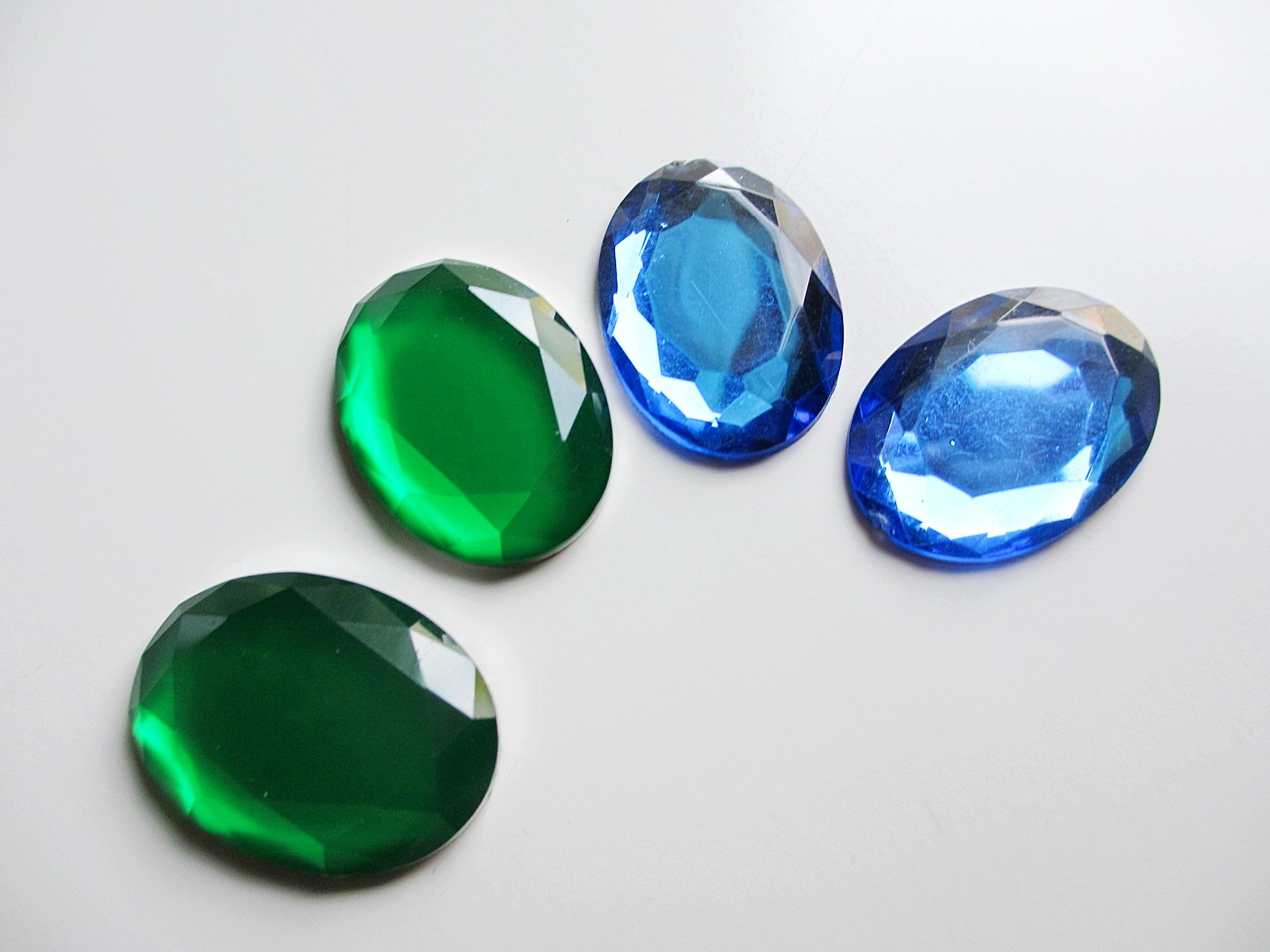In the image, four oval-shaped gemstones are arranged in an arched formation on a plain white background. Illuminated by light coming from the upper right-hand corner, the gemstones display a variety of vibrant colors and intricate facets that create a sparkling effect. Two of the stones are a rich green; the one on the far left is the darkest, resembling an emerald, while the other green stone is noticeably lighter. The remaining two stones are a striking blue, similar to aquamarines. Among these, the stone on the right stands out as the brightest, with stark highlights and visible surface scratches that contrast with its deeper blue hues. The interplay of light and color across the stones creates a captivating visual display.